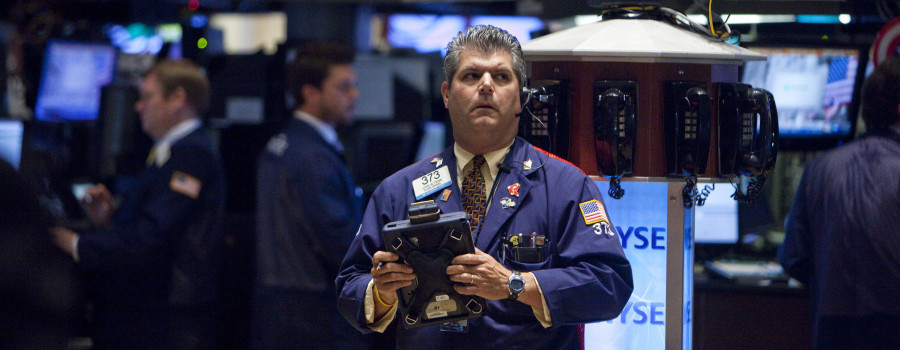In this image, we see a classic scene from the floor of the New York Stock Exchange, prominently featuring a stock trader with employee number 373. He wears a distinctive navy blue jacket that marries elements of both casual and sportswear. The jacket is adorned with multiple pins and boasts a United States flag patch on the left side, directly above his employee number. Beneath the jacket, he wears a crisp white shirt paired with a tie. On his left wrist, he sports a digital wristwatch, while in his right hand, he holds an electronic device fitted with a stylus.

The background adds depth to the bustling environment: a circular arrangement of black telephones is mounted on a cylindrical structure made of wood or plastic, ensuring accessibility for the traders. A sign beneath the telephones displays "NYSE," denoting the New York Stock Exchange. Other traders, similarly dressed in navy blue jackets, are visible but blurred due to the shallow depth of field, drawing focus to the central figure. The stock trader, characterized by grey hair and a round face, gazes intently to the left, encapsulating the intense atmosphere of the trading floor.